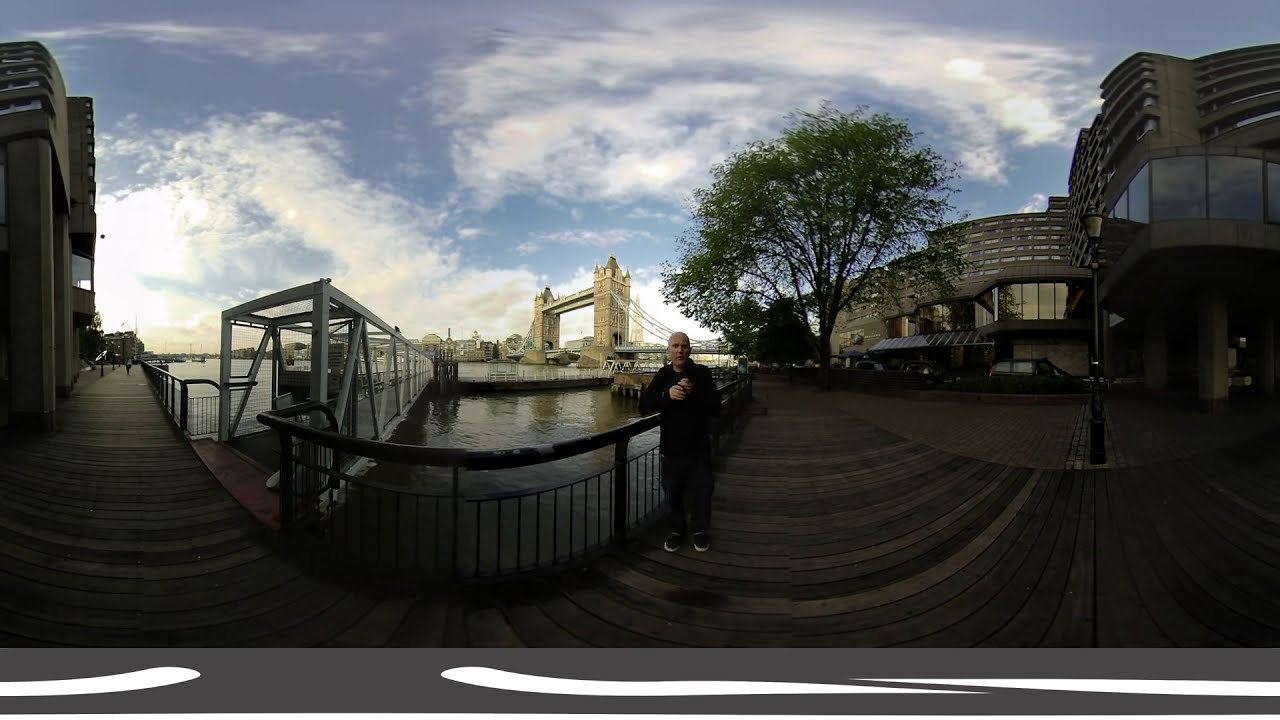A photograph captures a man standing on a wooden boardwalk by a river at dusk, with a sprawling, coffee-colored brown bridge dominating the background. The sky is a deepening blue, dotted with clouds, adding to the overall dimness of the scene. The man, who appears to be bald and dressed entirely in dark clothing, including a black hoodie, blue jeans, and black and white shoes, gazes directly into the camera. He holds something in his hand, although it's not clear what it is. To his left, the boardwalk wraps around the front and extends to the right, flanked by several buildings with see-through windows and adorned with a large tree full of green leaves. The area has a sophisticated yet lively feel, complete with lampposts, cars, and a small deck that might be used for boats, adding to the ambiance of a bustling cityscape, likely in England. The contrast between the massive, foreboding bridge and the serene river beneath it creates an intriguing backdrop for the man's contemplative stance.